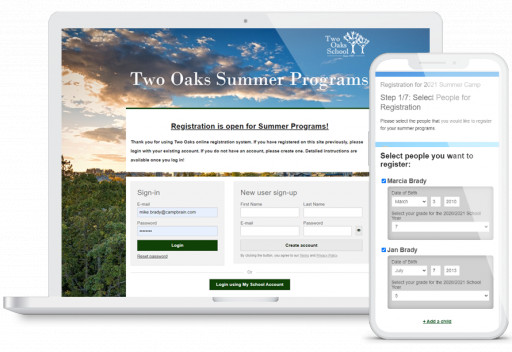A clean, modern header image features an iMac and an iPhone, both showcasing elements of a summer camp registration process. The iPhone display highlights step one of seven of the sign-up process, where users are prompted to select individuals for registration; Marsha Brady and Jan Brady are pre-selected. The screen exhibits a detailed interface with grey informational boxes possibly containing their date of birth and age. Meanwhile, the iMac screen shows a capture of the Two Oaks summer programs' website, with bold text announcing that registration is open for summer. The background of the website image displays a serene open field under a partly cloudy sky. Both devices are set against a plain white background with subtle drop shadows, giving a clean and professional representation of the registration process.